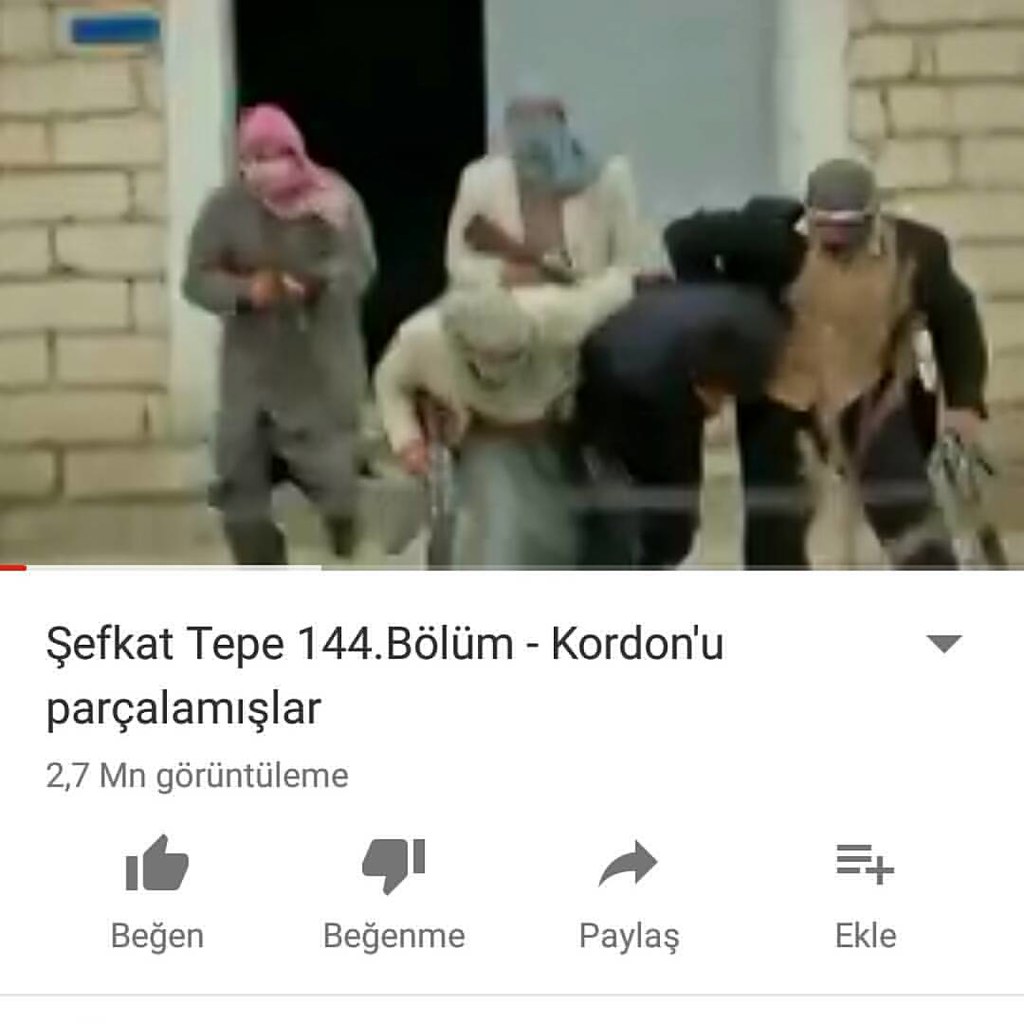The image depicts a social media post showing a blurred photograph of a potentially violent scene involving a group of men and a hostage. The photograph appears to be taken from a computer screen, and is partially obscured by a colorful lower section with text reading "Sefkat Tepe 144 Balaam Dash Kordanyu Parkala Mislar," which also includes typical social media interaction icons such as thumbs up, thumbs down, and share buttons. The text beneath this section is in an unidentified foreign language. In the image, the men are wearing various outfits and headscarves, some resembling bandanas or towels, while holding the hostage, who is dressed in a dark suit and crouching. The men are equipped with guns, possibly automatic weapons, and their attire includes gray with a pink head covering, lighter clothing, and a dark suit with a tan shirt. The exact nature of the scene—whether it is a depiction of hostage-taking or a rescue operation—is unclear.